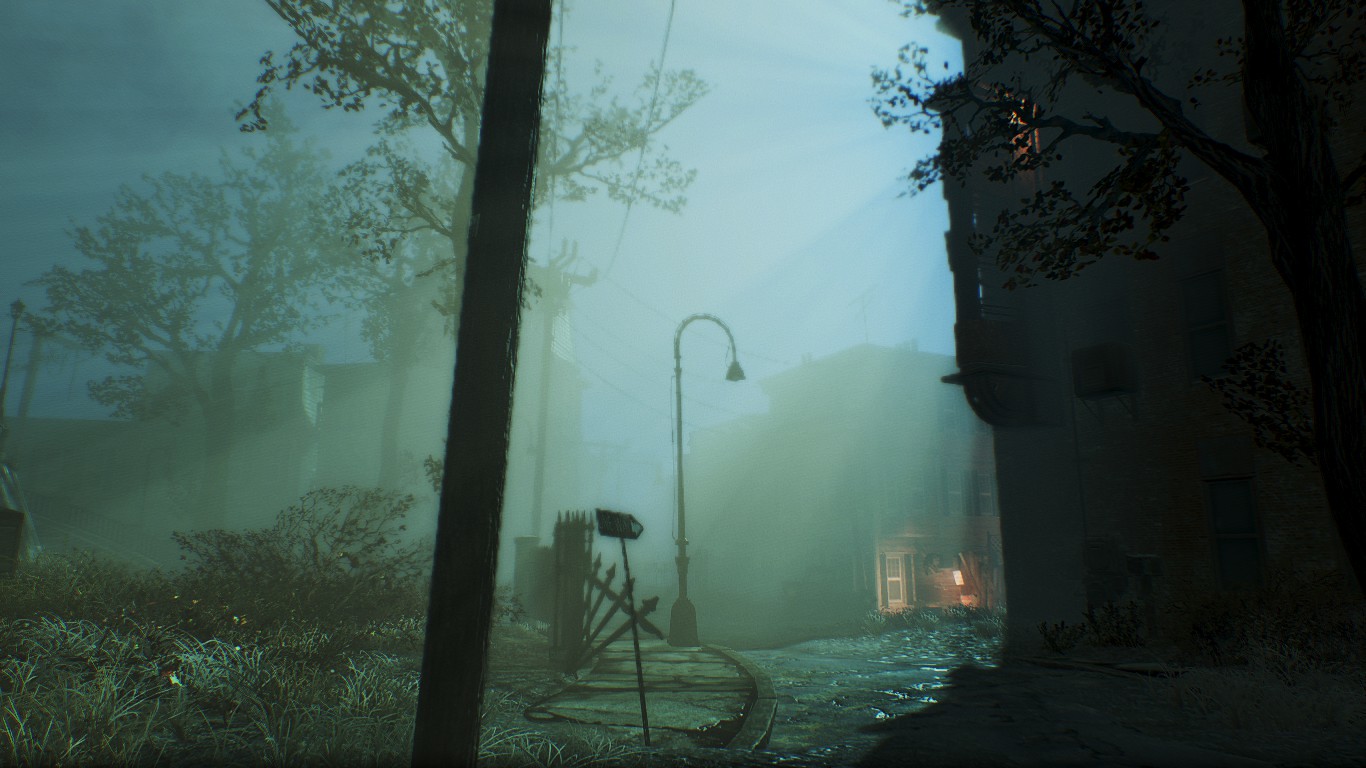The image, likely AI-generated, depicts an eerie, fog-covered street at night, evoking a scene from an abandoned town or a spooky video game. The sky is a deep, dark blue, with moonlight barely visible, casting disorienting shadows. In the center, an old, non-functioning streetlamp with a U-shaped, umbrella handle design stands near an uneven, ancient-looking cobblestone sidewalk. 

On the right side, a dilapidated house seems to emerge from the mist, partially obscured by shadows. A patio, though unclear and shrouded in darkness, hints at neglect. One upstairs window emits an amber or red light, making the scene even more haunting. A crooked tree with sparse leaves stands ominously in front of the house, contributing to the scene's ghostly ambiance.

Additional elements include a partially collapsed fence almost touching the sidewalk and a peculiar telephone pole with a missing trunk, obscured by an oddly placed electrical pole. To the left, more trees stand as dark silhouettes, adding to the spooky atmosphere, while brown, withered bushes and a random bird feeder accent the eerie setting. The entire street appears wet and shiny, enhancing the sense of abandonment and decay.